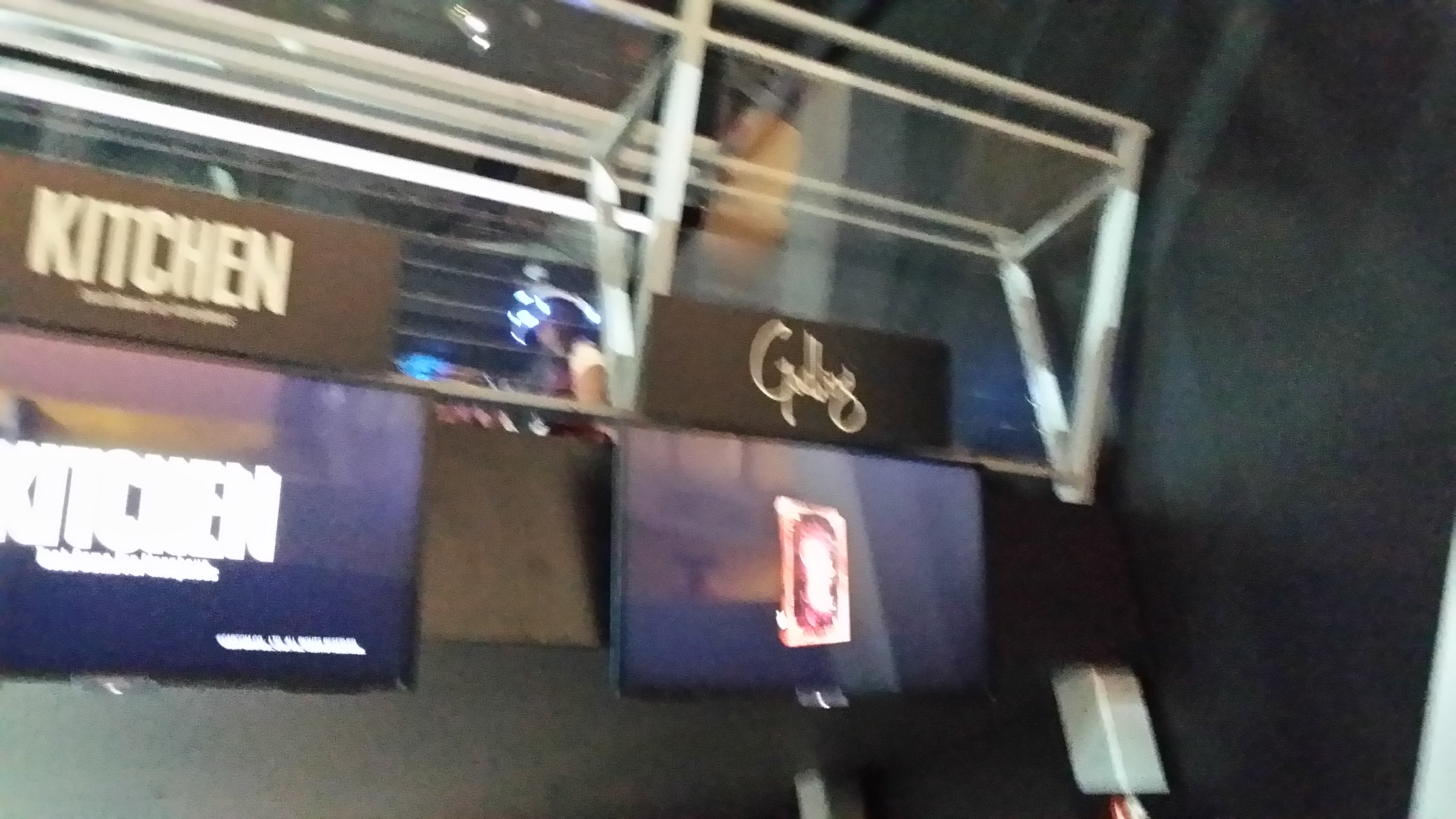The image depicts a series of signs mounted on an overhanging wall, characterized by a grayish background color. The wall extends to the right-hand side where a small light gray box can be seen at the bottom right corner. Central to the image are two flat-screen TVs; the one on the left displays very blurry white text reading "Kitchen," while the screen on the right features a design incorporating white and pink elements. On the left-hand side of the image, there is a sign with a dark brown background and white text that also reads "Kitchen." The right-hand side showcases another sign with white cursive text. Above these signs, a series of light gray and white railings add a structural element to the composition, completing the overall scene.